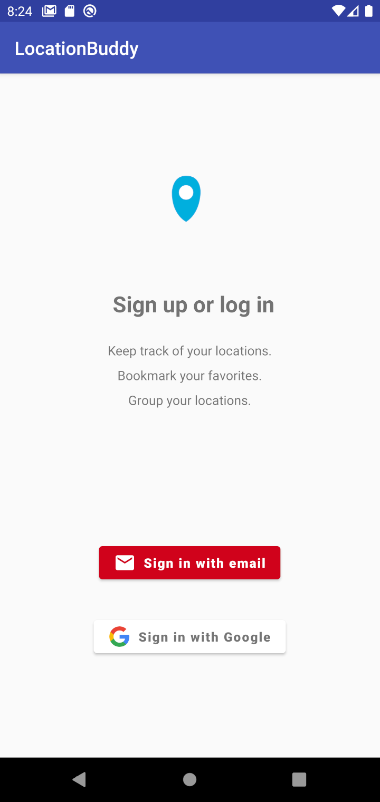A mobile screen capture displays the interface of the "Location Buddy" app. The top bar shows a time of 8:24 on the left, accompanied by icons indicating mail, an SD card, Wi-Fi, signal strength, and a fully charged battery (100%). The background is vividly blue, segmented into various sections.

The app’s title, "Location Buddy," is prominently displayed at the top in white text. Below it is a light gray screen with a blue pin icon in the center. The interface prompts the user to "Sign Up" or "Log In," emphasizing the app's features: keeping track of locations, bookmarking favorites, and grouping locations.

A prominent red button with white text encourages users to "Sign in with Email," featuring a small envelope icon to its left. Beneath it, a white button with black (or dark gray) text offers the option to "Sign in with Google," adorned with the familiar Google "G" logo.

At the very bottom, standard navigation icons are present: back, stop, and a circular button that suggests access to the menu.